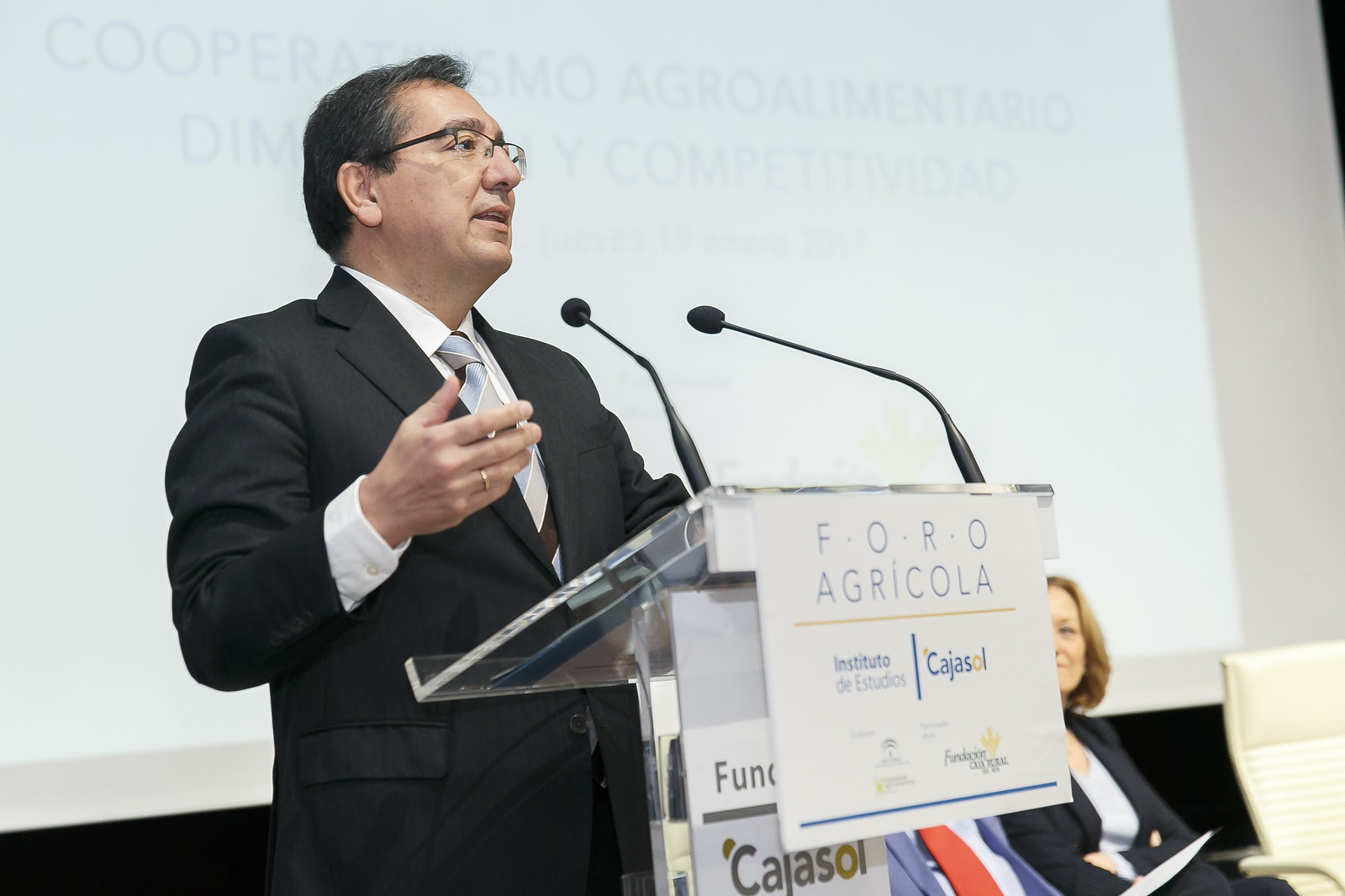A man, slightly on the heavier side, stands at a clear acrylic podium, likely made of glass or thick plastic, equipped with two small microphones. He is dressed in a black suit with a white button-down shirt and a tie featuring wide stripes in varying shades of silver, blue, gray, taupe, and brown. His thin, rimless glasses have black earpieces. With dark brown to black hair, lightly streaked with gray, he looks to his left at the audience. A wedding band is visible on his expressive right hand. The podium displays a sign reading "F.O.R.O. Agricola, Instituto Estudios Cajasol." To his right, a woman in a black suit and light blue-to-white shirt sits, her face partially obscured. Another person, mostly hidden by the placard, is seen wearing a grayish-blue suit with a red tie and a light blue shirt. Behind the speakers, a projector screen shows faint, illegible Spanish text, including partial words such as "Cooper, Agro Elementario." The scene suggests an agricultural forum, possibly in South America.